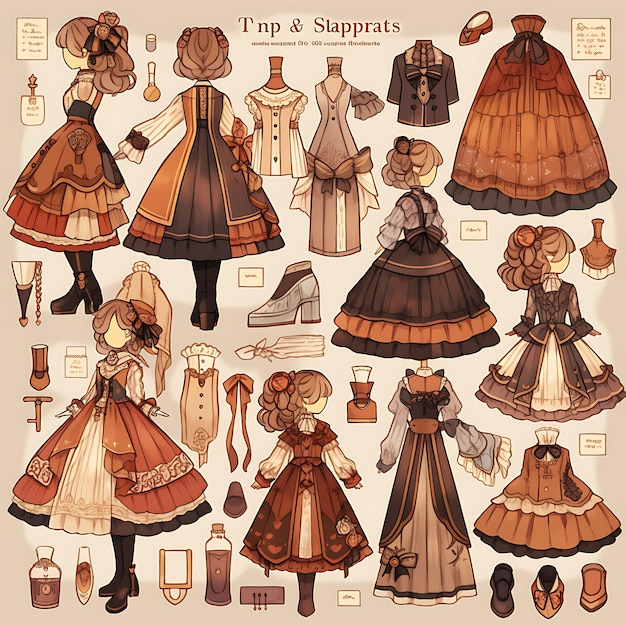The image features a character model sheet with various Victorian-era dresses and accessories depicted in an anime-style cartoon. The background has a tan hue, creating a sepia-like effect, and the color palette includes browns, tans, reds, whites, blacks, and golds. There are faceless mannequins modeling at least six different dresses, each shown from multiple angles including the front, back, and sides. The dresses are multi-layered with ridges and frills, and range from different shades of red to grey and white. Additionally, the sheet includes shoes, high heels, ribbons, bows, and bottles of fluid, all scattered without a specific order. At the top of the sheet, there are handwritten labels including "T," "NP," and "slap rats". A small girl with curly brown hair adorned with a flower is also visible, modeling some of the dresses from behind. Overall, the image resembles a detailed and whimsical diagram of historical fashion.